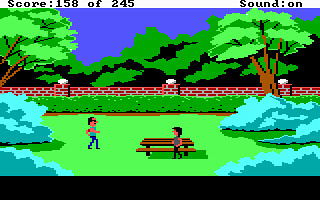The image is a small, widened screenshot, about a quarter of the usual viewing size, with a 15% black letterbox at the bottom. Above the image, a white background displays a score of "150 of 245" on the left and "sound: on" on the right. The image itself, reminiscent of the pixelated, blocky graphics of an old Nintendo, Atari, Commodore 64, or Apple IIe game, depicts a park scene. In the center, there is a person sitting at a picnic table, while another stands to the left, approaching. The background features a purple sky, a hedge in front of a brick wall, and trees lining the scene on either side. The visual style gives a retro, digitalized feel to the setting.